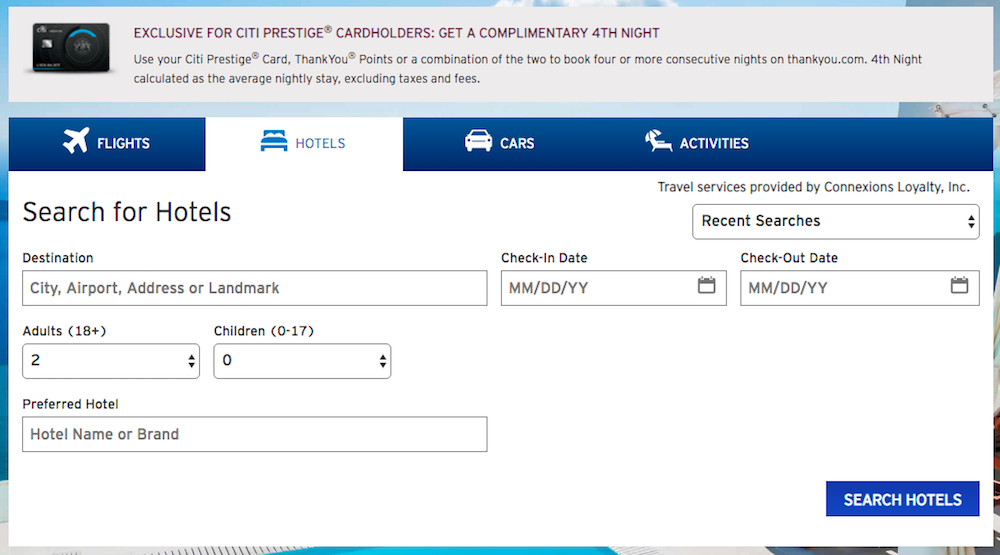**Detailed Caption for the Hotel Booking Interface Image:**

The image displays an online hotel booking interface with multiple functionalities. At the top, there's a gray bar featuring a credit card icon accompanied by the text: "Exclusive for Citi® Prestige Cardholders - Get a complimentary fourth night. Use your Citi® Prestige Card, ThankYou® Points, or a combination of the two to book four or more consecutive nights on ThankYou.com. The fourth night is calculated as the average nightly rate, excluding taxes and fees."

Below this, the interface is structured with tabs for different travel services. 

1. **Tabs Overview**:
   - **Hotels Tab**: Active, highlighted in blue with a white bed icon and blue text.
   - **Flights Tab**: Located to the left, with a blue background, white airplane icon, and "Flights" written in white.
   - **Cars Tab**: Shows a white car icon and "Cars" text on a blue background.
   - **Activities Tab**: Displays a beach chair and umbrella icon in white with "Activities" text on a blue background.

2. **Hotel Booking Section**:
   - Next to the tabs, there’s a section labeled "Search for hotels."
   - To the far right, under the gray bar, it says "Travel services provided by Connections Loyalty Inc."
   - Below this, there is a "Recent Searches" section with up and down arrows to navigate through previously looked-up destinations.

3. **Booking Form**:
   - **Destination**: A text box labeled "Destination" where the user can type in a city, airport, address, or landmark.
   - **Check-in Date**: A calendar picker for selecting the month, day, and year of check-in.
   - **Check-out Date**: Similar to the check-in date, with its own calendar picker for the check-out date.
   - **Guests**:
     - **Adults (18+)**: An adjustable number input with up and down arrows, currently set to 2 adults.
     - **Children (0-17)**: Another adjustable number input for the count of children, currently set to 0.
   - **Preferred Hotel**: A text box for typing in a specific hotel name or brand.
   - **Search Hotels Button**: A blue button with white text located at the bottom right corner to initiate the search.

All these elements are displayed against a clean white background with black text for easy readability.